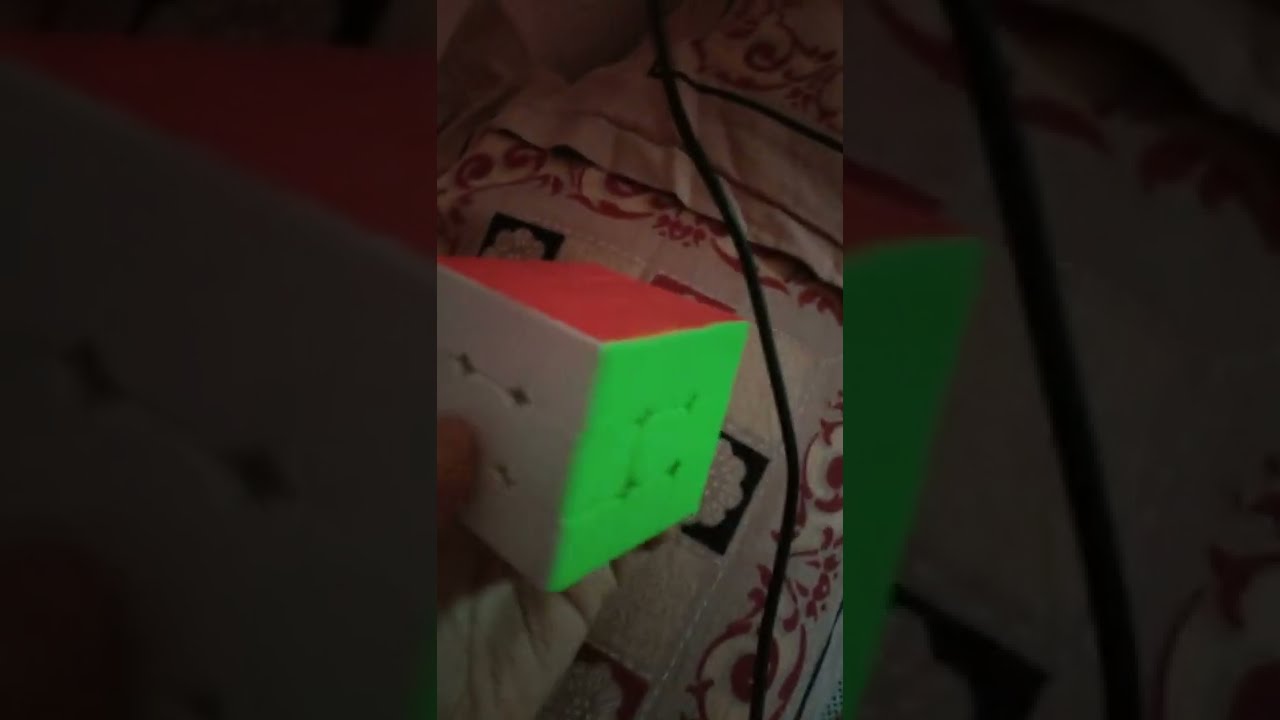This color photograph features a close-up of a man holding a Rubik's Cube which has been solved, revealing an all-white side where his thumb rests. The top of the cube is predominantly coral-colored, while the left side is white and the right side shows a green surface. The cube is held above a vibrant blanket adorned with intricate floral embroidery, showcasing blue, red, and other colorful flowers, leaves, and vines. The image is split into three panels; the central panel is crisply detailed, focusing sharply on the man's hands and the Rubik's Cube. In contrast, the left and right panels offer blurred, darkened close-ups of the main scene, drawing clear attention to the well-lit, central image while subtly highlighting the blanket’s elegant yet somewhat juvenile design. A black wire runs across the blanket, adding a subtle contrast to the colorful and detailed background.